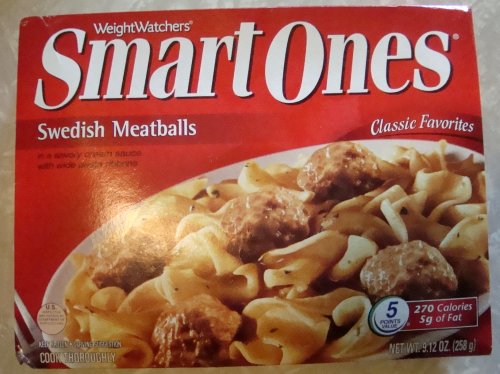This color photograph captures the front of a food packaging, likely a carton or box, set against a gray background. The majority of the packaging features a vivid red backdrop adorned with white text. At the top, prominent branding reads "Weight Watchers" followed by the product name, "Smart Ones, Swedish Meatballs, Classic Favorites." 

The central and lower portions of the package highlight an appetizing depiction of the meal: golden pasta paired with brown Swedish meatballs, all served in a bowl. Light from above casts a gentle glow on the left side of the dish, enhancing its appeal.

In the bottom right corner, a circular logo with the number "5" inside is visible. Adjacent to this, a rectangular label in white text announces "270 calories" and "5 grams of fat." Below this nutritional information, faint white text indicates the product's weight.